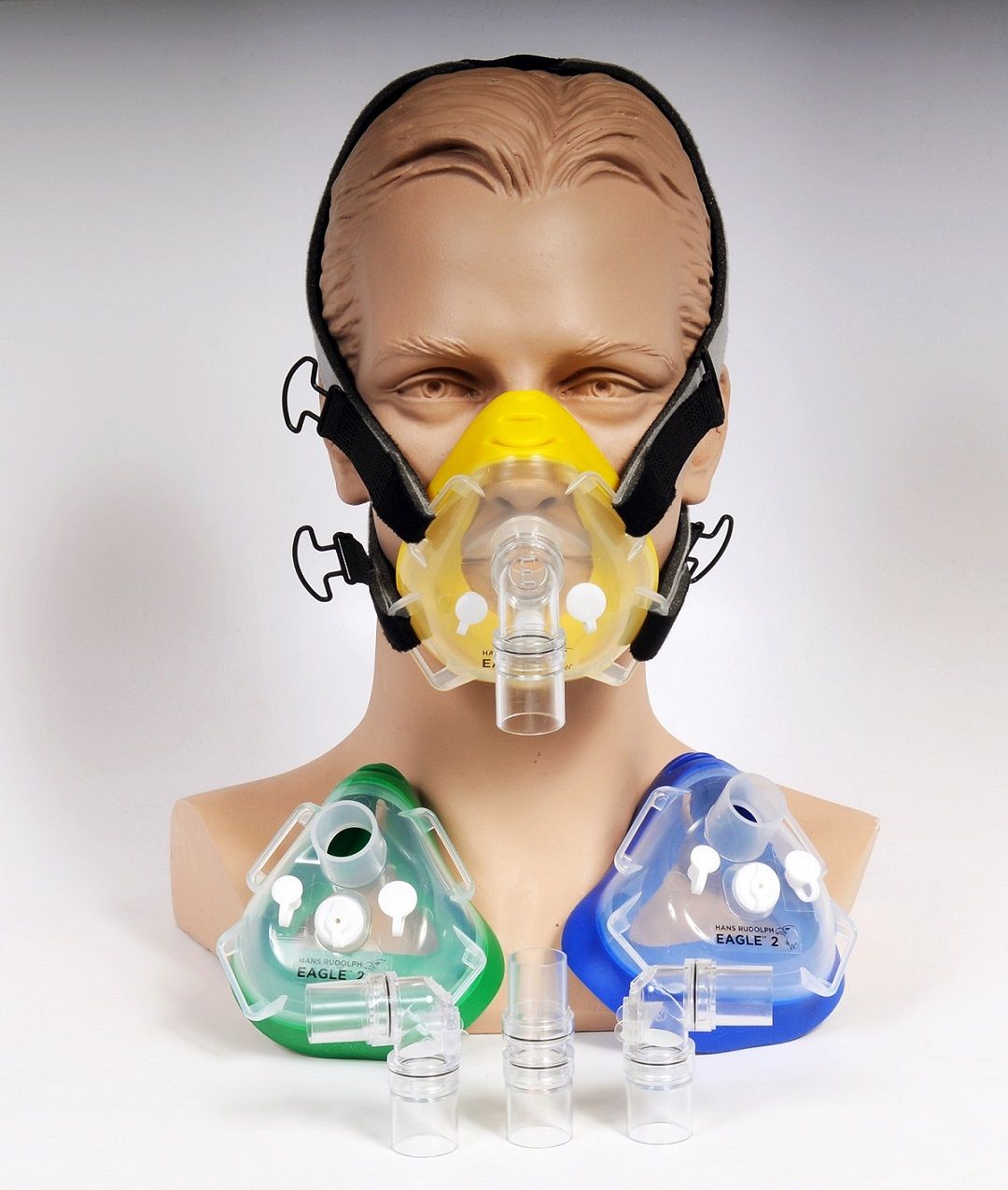The image prominently features a lifelike, albeit eerily realistic, mannequin bust used for demonstrating respiratory masks. The bust extends down to the shoulders, cut off at the chest, with unsettlingly artificial eyes that match the mannequin's flesh tone. Affixed to the mannequin's face is a yellow gas mask, secured with black straps, featuring a clear, unconnected tube. Additionally, there are two more masks positioned below the bust—one green and one blue—both labeled with the title "Eagle 2" and accompanied by several clear tubes.